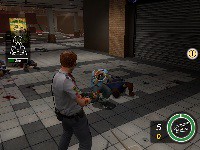The screenshot from the video game appears to be quite small and dark, making details somewhat challenging to discern. The scene is set in a garage-like environment, characterized by a visible garage door in the top right corner. The floor is tiled with a mix of light and dark gray squares, and brick walls are noticeable in the background. The central character, likely a white male, is seen from behind, dressed in a gray or white shirt and dark pants, with a gun aimed at an adversary, possibly an animal or creature, ahead of him. Indications suggest this is a third-person shooter game, given the perspective from which the character is viewed. The interface includes a prominent red and blue crosshair targeting the enemy, whose health bar, nearly depleted, is shown in green at the top left. The bottom right corner displays a green circle with a nearby '5', likely indicating the ammo count, accompanied by a '0' below it. Additionally, an emblem resembling a Christmas tree appears in the background, adding to the intricate details of the game's setting.